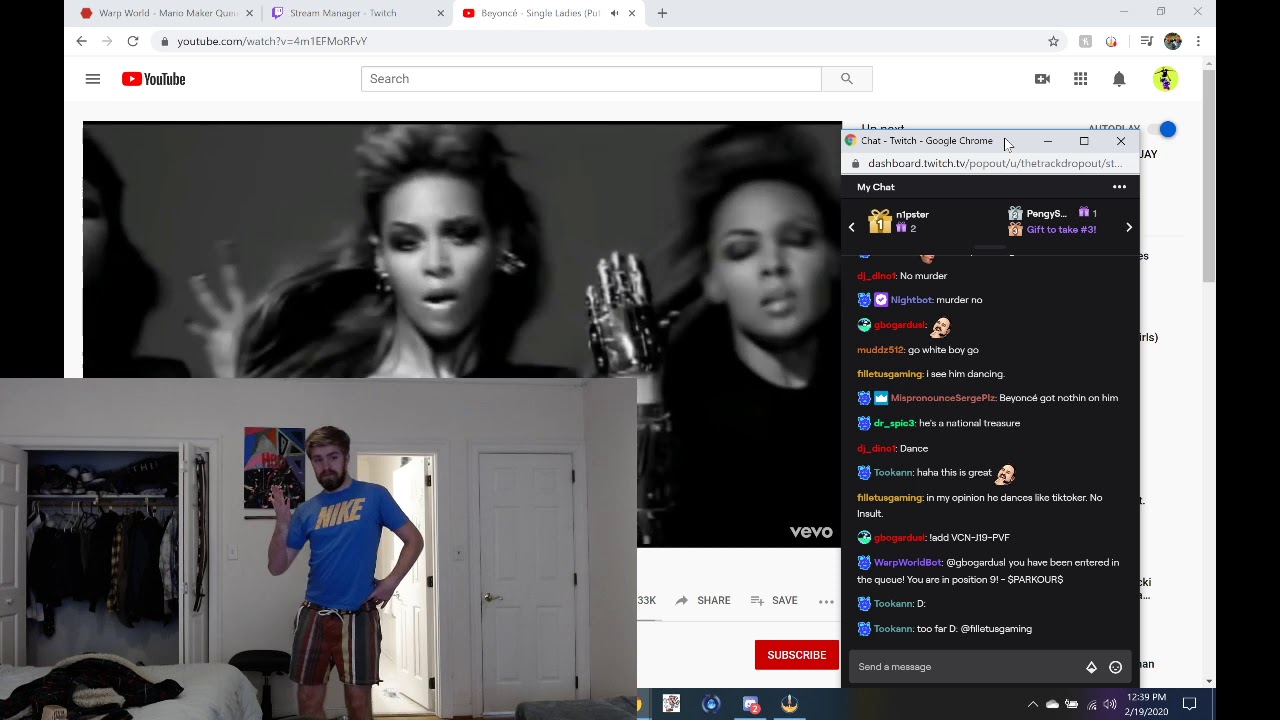At the very top left corner, the screen shows "Warp World Mario Maker Stream Manager" for Twitch. Below it, there is a video titled "Beyonce - Single Ladies (Put a Ring on It)" with the YouTube URL: youtube.com/watch?v=4m1EFmRF3eY. The interface includes a gray-colored hamburger menu, a YouTube search bar with a gray question mark, a camera icon, a grid of nine dots, and a bell icon. 

On the screen, the Twitch chat is visible, and the webpage is opened in Google Chrome. The stream features someone performing the "Single Ladies" dance made famous by Beyonce. The person is standing up with one hand raised and the other hand on their hip, mimicking the dance moves. The background includes a white wall, an open door, and a closed one, as well as a bed.

The timestamp on the video shows 12:30 PM on February 19, 2020. The chat includes various comments, but notably lacks any mention of the word "murder." The participant’s dancing style is compared to TikTok dances, with some viewers commenting positively. 

An on-screen notification reads "You have entered the queue. You are in position ID too far." Another comment suggests a feeling of being scammed, indicating some viewers shared mixed reactions to the stream.